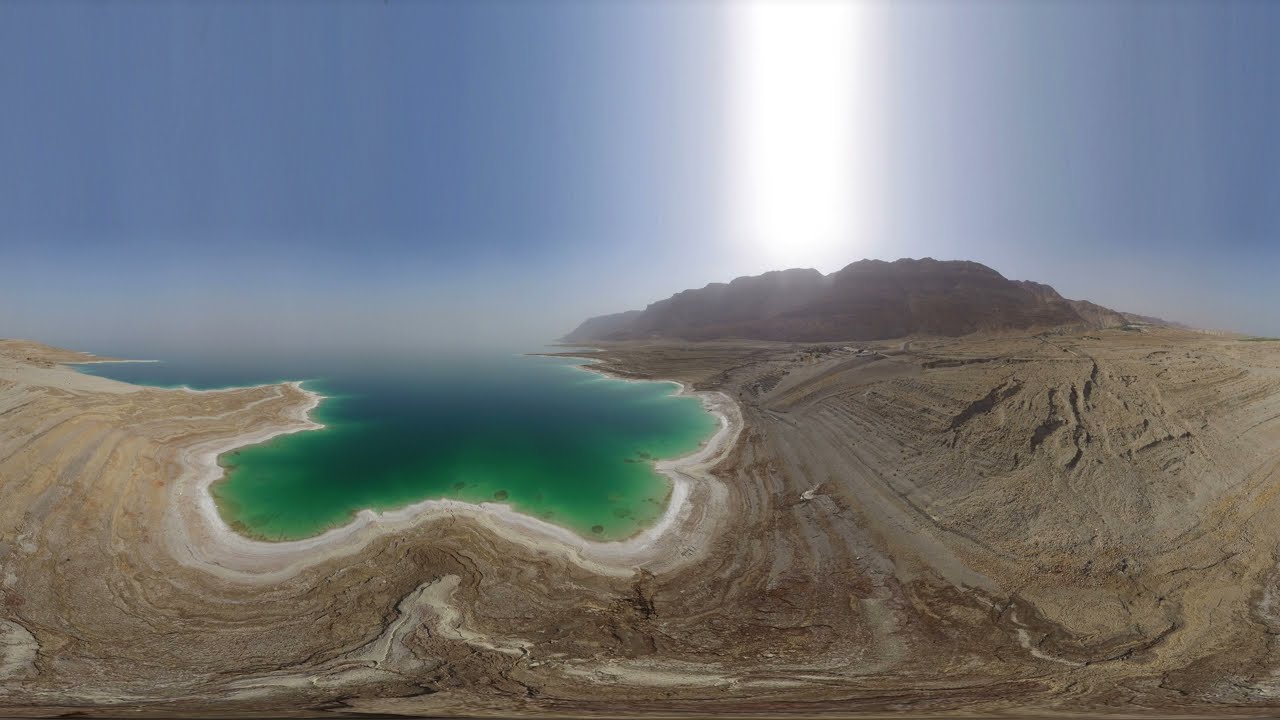This striking aerial photograph, possibly taken with a GoPro or created digitally, captures a mesmerizing desert oasis. A stunning, curved landmass of brown mud and sand features deep crevices and layers that ripple outward. Nestled between this rugged terrain lies a body of water with vivid green edges transitioning to dark blue in the center, giving it an almost otherworldly glow. Surrounding the lake is a striking white outline, irregular in shape. Rising above the landscape, sheer rock cliffs and distant mountains frame the scene, topped by a clear blue sky. A brilliant vertical cone of sunlight beams down from the right of center, illuminating the mud, sand, and water with a celestial quality. The seamless blend of natural and possibly computer-generated elements creates an image that is both beautiful and surreal.